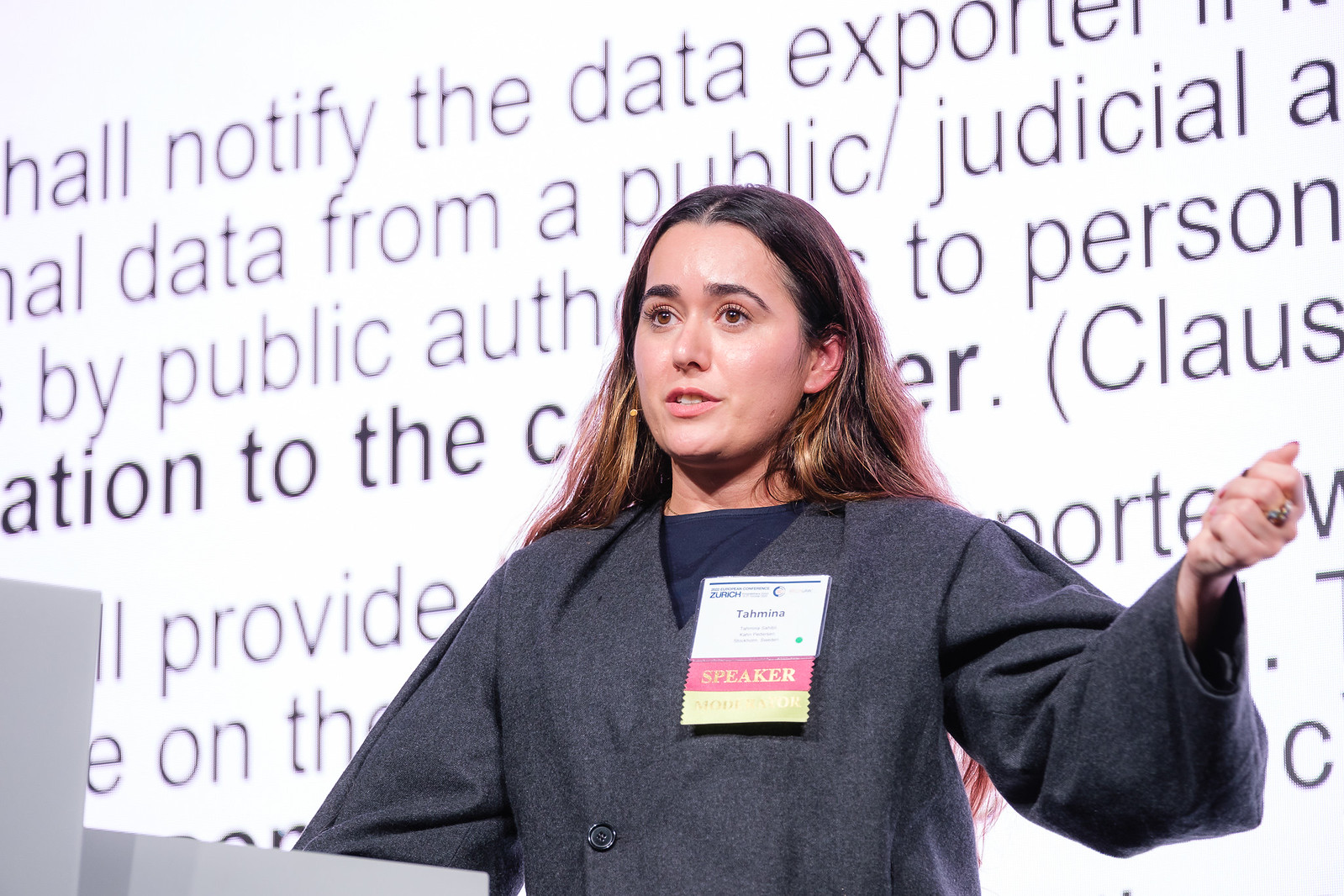The image features a young woman named Tamina, who appears to be in her 30s, standing at a gray podium at what seems to be a technical conference or convention. She has long black-brown hair, brown eyes, and is dressed in a gray blazer over a navy blue top. Tamina is wearing a name tag that identifies her as a speaker, adorned with both a red ribbon labeled "Speaker" and a gold ribbon likely saying "Moderator." She is positioned to the front right of a large screen displaying a slideshow with the text "shall notify the data exporter" and "data from a public/judicial." The words on the presentation are black on a white background. Tamina's right hand is raised in the air, with her fist clenched as though she is making a point.